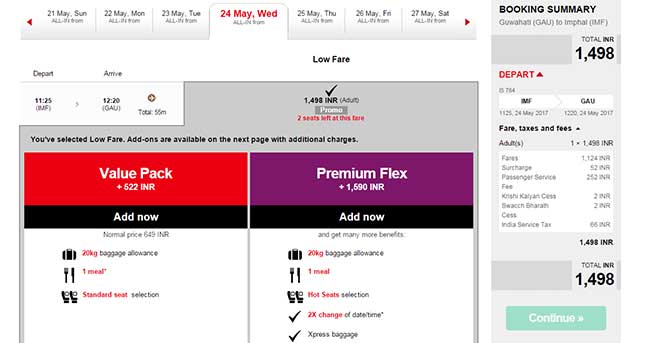The image depicts an airline reservation webpage, detailing options for booking a flight from Guwahati to Imphal. Spanning the top of the page are tabbed dates from Sunday, May 21st to Saturday, May 27th, with Wednesday, May 24th prominently highlighted. Beneath these tabs, a section indicates available low-fare options, showing that an adult fare is priced at 1,498 INR, with only two seats left at this rate.

Below, there are prompts about add-on packages that can be included on the next page. One such option is the Value Pack, costing an additional 522 INR, which includes 20 kg of extra baggage, one meal, and a standard seat. Another option is the Premium Flex plan, priced at 1,590 INR, which offers 20 kg of extra baggage, one meal, priority seating, the ability to change date and time twice, and express baggage service.

On the far right, a booking summary recaps the selected options: the departing city (Guwahati), the destination (Imphal), the flight cost (1,498 INR), the chosen date (May 24th), and various fare breakdowns that include surcharges, passenger charges, and an Indian service tax. Users are then given the option to proceed with booking the flight.